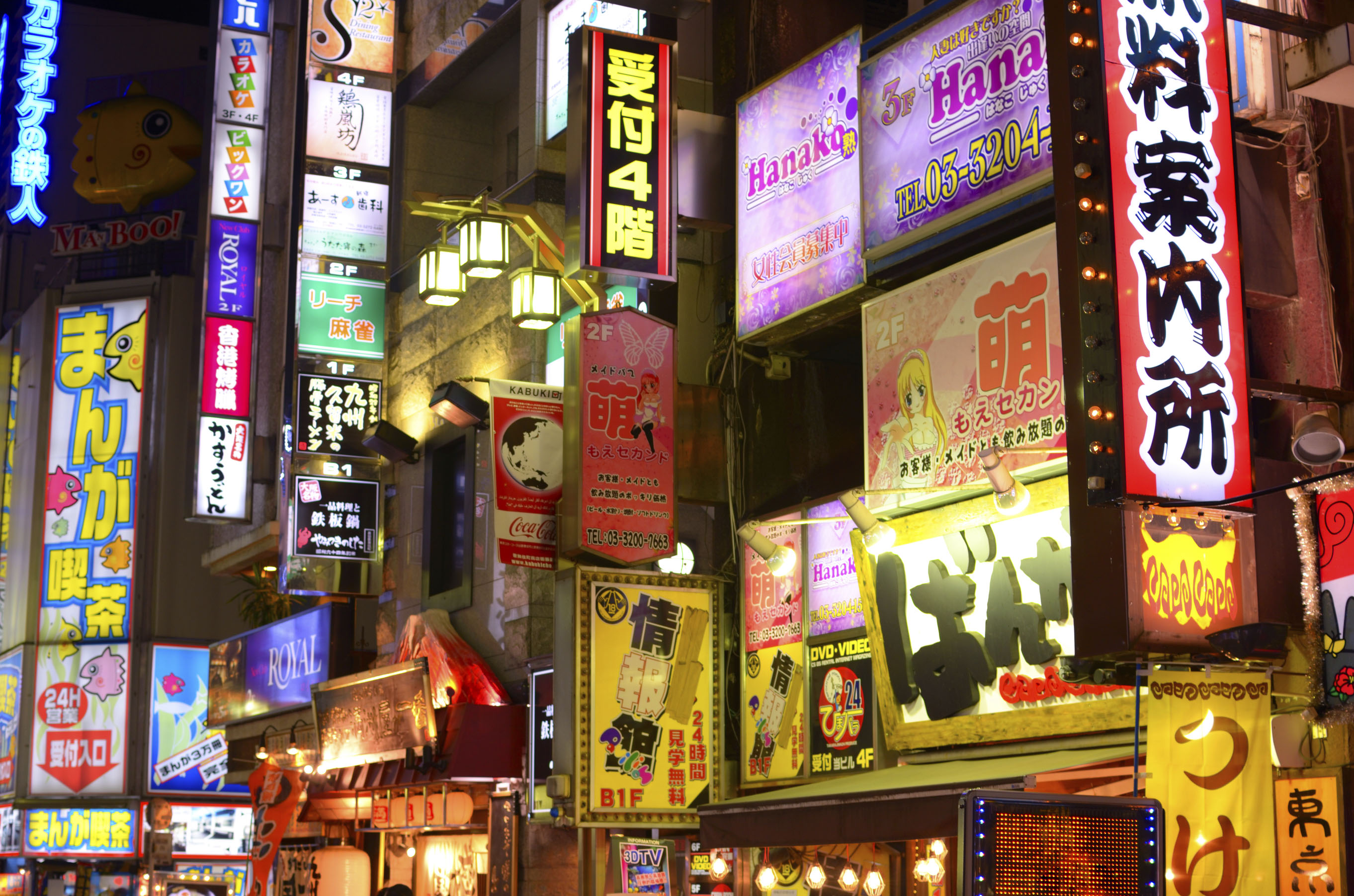The image depicts the bustling upper facade of a street in an Asian community, likely a Chinatown, adorned with a dense array of vibrant advertisements and signs in various Asian scripts. Dominating the view are vertical and rectangular billboards in a spectrum of colors: red with black characters, purple with "Hanako" spelled out, and multiple others in white, blue, yellow, and pink hues. A standout feature includes a Pikachu-like character atop a billboard to the left. Hanging lamps or street lights dangle over the scene, adding to the lively atmosphere. The bottom frame captures the tops of storefronts, all contributing to a tightly packed display of commerce and culture.